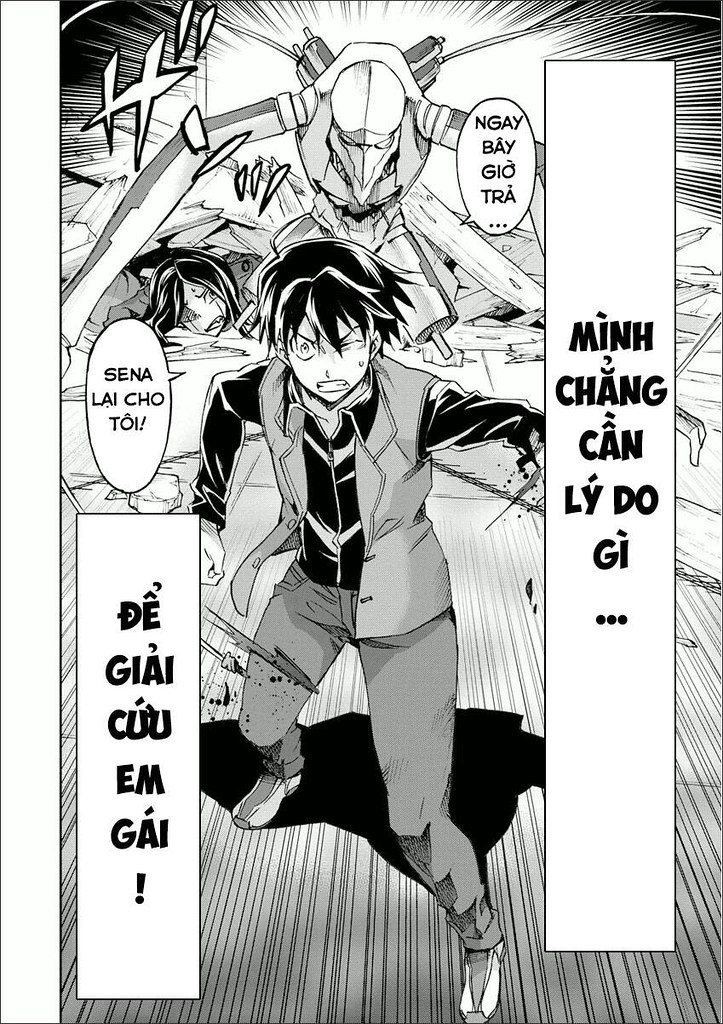This vertically aligned, black-and-white comic strip image features a dramatic encounter between a central character and a menacing robotic creature. The scene is rendered in an anime style, characterized by precise linework and expressive details. At the top of the image, a fearsome, mechanical monster with long arms, a masked head, and possibly wings, appears to be chasing the person in the center. The central character, wearing a gray vest over a black shirt with gray pants, has a strained expression with wide eyes, spiky short black hair, and an angry look on their face as they glance back at the creature.

To the left of this character, a speech bubble with the exclamation "Sina Le Cho Toi!" (L-A-I-C-H-O-T-O-I) indicates a heightened sense of urgency or danger. The robotic pursuer on the right side of the image shouts "N-G-A-Y-B-A-Y-G-I-O-T-R-A," further escalating the tension. Beneath the creature, partially obscured by rubble, lies a figure who appears to be badly injured or possibly dead, adding to the scene's intensity.

Flanking the lower part of the image, there are vertical, bolded black strips of text. On the left, it reads "D-G-I-Q-M-G!" whereas the right side states "Min Chang Kan Lee Do Ji," alluding to the ongoing drama. The use of different shades of gray enhances the depth and mood of this captivating and tense comic scene.